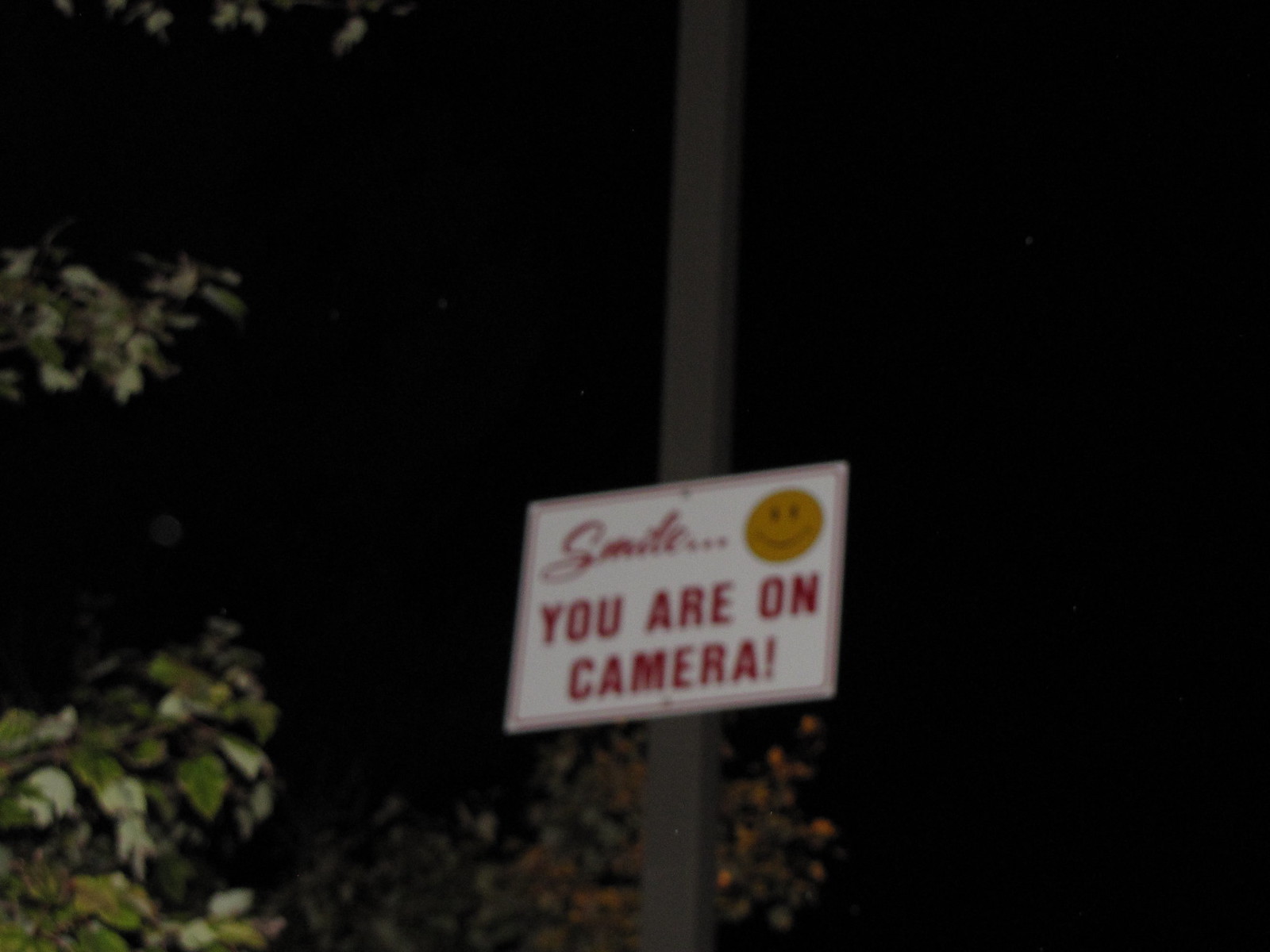This nighttime photograph captures a tall, square metal pole standing outdoor. Affixed to the pole is a sign with cheerful text and imagery. The sign features the word "Smile" followed by three dots and a yellow smiley face emoji. Beneath this, in bold, capital letters, it reads, "YOU ARE ON CAMERA!" The background reveals a natural setting, with leaves and branches visible on multiple sides of the pole. On the left side, leaves protrude from the top corner, a solitary branch extends out from the middle, and a cluster of leaves occupies the bottom left corner. Additionally, in the center bottom part of the image, more limbs, adorned with yellow leaves, extend upward, adding rich foliage detail to the scene.